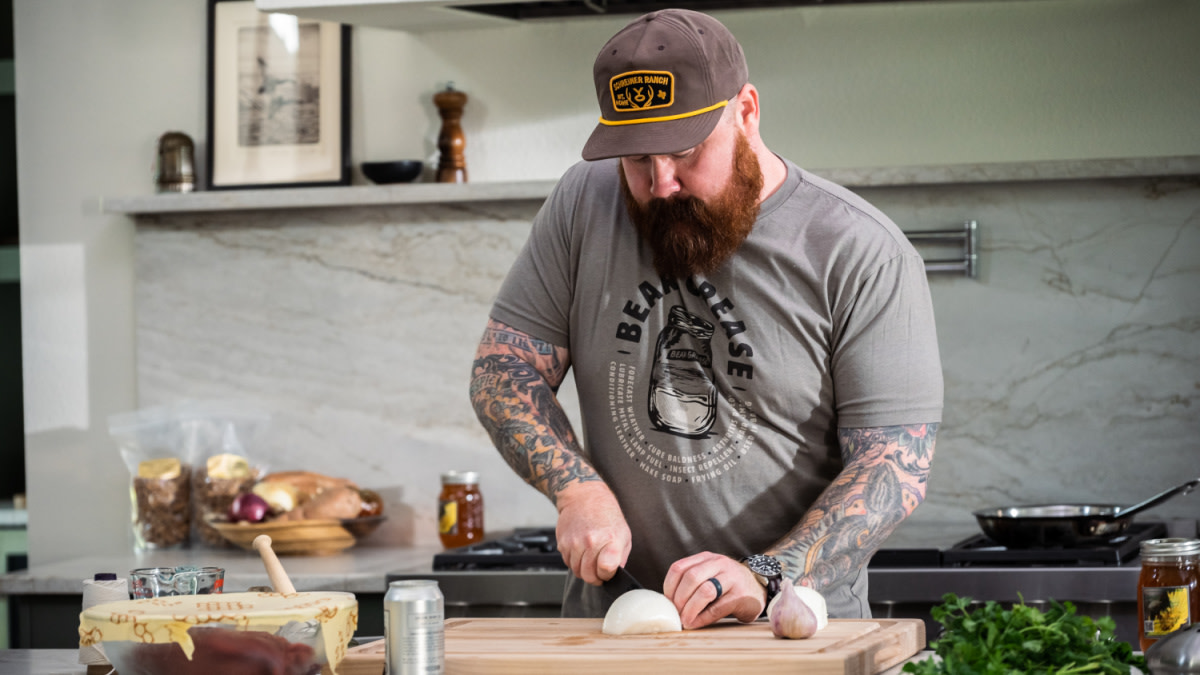The photograph depicts a man, likely Kevin from Top Chef Las Vegas, in a kitchen engaged in preparing food. He has a distinctive thick red beard and is wearing a gray shirt adorned with text and imagery, accompanied by a brown hat with yellow accents. His heavily tattooed arms are visible below short sleeves, and on his left hand, he sports both a watch and a black wedding ring. The man is focused on chopping a white onion on a wooden cutting board. In front of the board lies a can of beer, and to its left, a bowl covered with yellow plastic wrap, possibly containing a spoon. To the right of the cutting board is a bunch of parsley, also referred to as greenery, and a jar of what might be honey-colored preserves. Behind him stands a large stove with a frying pan resting on top, against a marble backsplash.